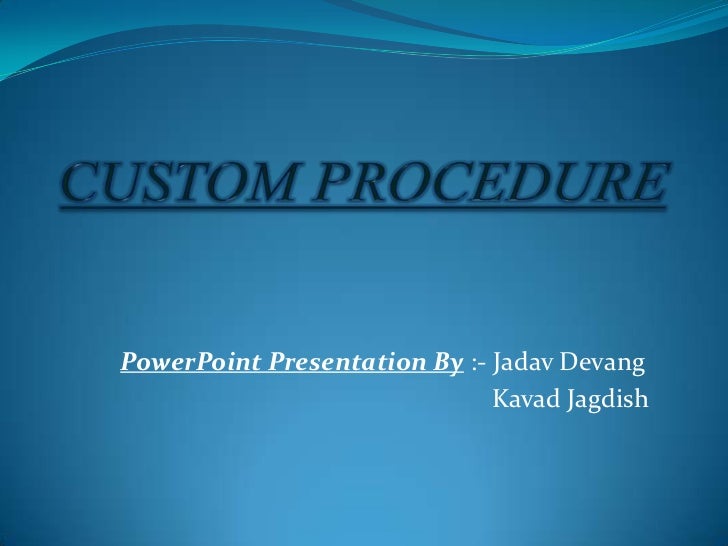The PowerPoint slide features a predominantly blue background with a lighter blue wave pattern at the top, transitioning into a gradient that lightens toward the center. Across the top third of the slide, large, black, capitalized, italicized, and underlined text prominently displays the title "Custom Procedure." Beneath this, about two-thirds down the slide, smaller white italicized text reads "PowerPoint Presentation by: Jadav Devang." Directly below this, in the same white text, the name "Kavad Jagdish" is listed. The design is cohesive, with the wavy pattern and text formatting providing a visually appealing and professional look.